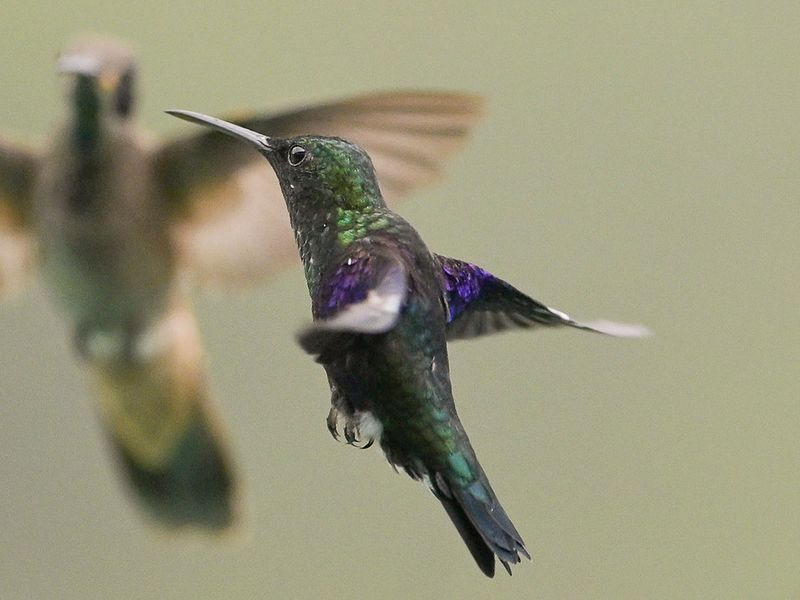In this vivid image, the foreground features a brilliantly detailed hummingbird in mid-flight. Its head displays a stunning iridescent green, transitioning into purple at the shoulders and the base of the wings. The bird's wings, captured in motion, shift from purple near the body to a darker black hue towards the tips, and are distinctly visible despite their rapid flutter. A long, grayish-black, needle-like beak and prominent black eyes define its face. The body of the hummingbird exhibits a greenish tone with touches of black, and its tail feathers mirror these darker shades, while its claws are a muted blackish-gray. The background contrasts sharply with the vivid hues of the foreground bird, presenting a light, matte, beige-gray color. In the background, a larger, blurred hummingbird hovers with outstretched wings, displaying a muted palette of browns, greens, and yellows.